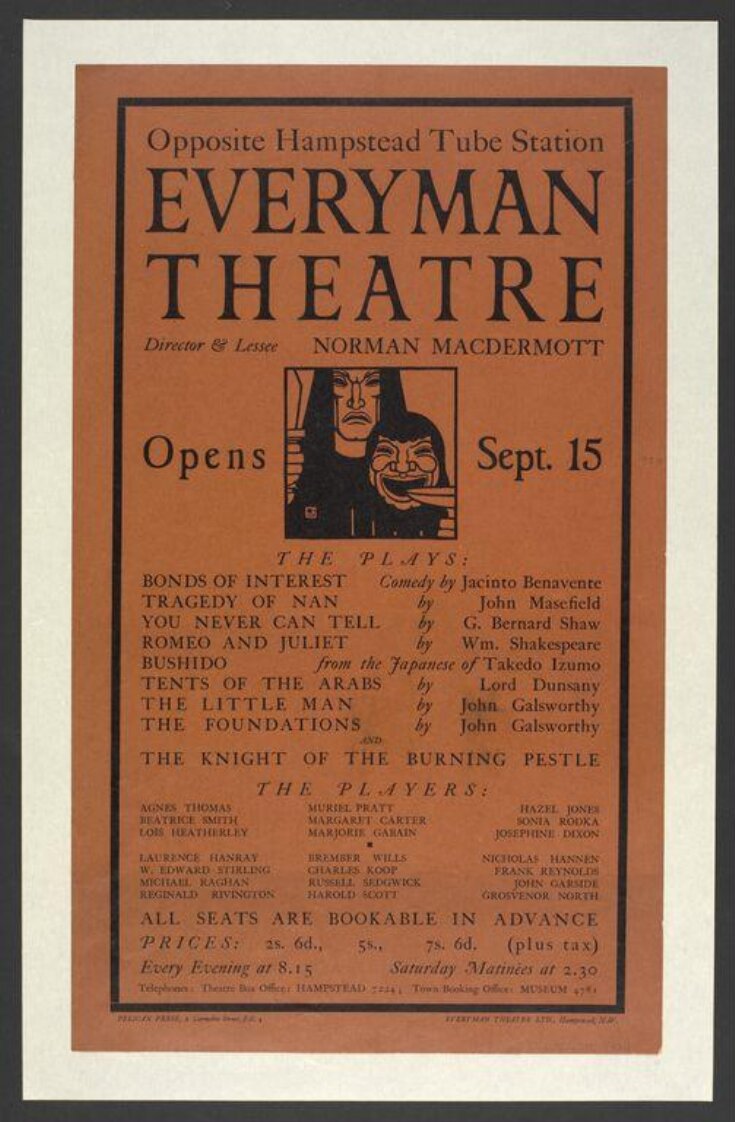This image is a portrait-oriented, black-and-white poster, framed with a black border and a white or cream-colored matte. The poster itself has a black rule about an inch inside the edge. It appears to be an advertisement for the Everyman Theatre, located opposite Hampstead Tube Station, and highlights its upcoming theater productions. At the top, the black text reads "Opposite Hampstead Tube Station," followed by larger, all-caps black text announcing "Everyman Theatre." Below, in smaller text, it mentions the director, Lacey Norman McDermott, and the opening date of September 15th.

Central to the poster is a square black-and-white illustration depicting two masked figures: a man on the left, frowning with long black hair, holding a knife, and another person on the right with a rounder face, smiling broadly. One of the masks depicted appears to have a wide-open mouth and squinty eyes, giving it a somewhat eerie look.

The poster continues to list several plays scheduled to be performed, including "Bonds of Interest," "Tragedy of Nan," "You Never Can Tell," "Romeo and Juliet" by William Shakespeare, "Bushido," "Tenets of the Arabs," "The Little Man" by John Galsworthy, "The Foundations," and "The Night of the Burning Pestle." It also features the names of notable playwrights such as Jacinto Benavente, John Masefield, Bernard Shaw, and John Galsworthy. Additional information at the bottom indicates all seats are bookable in advance, alongside pricing details. The overall style of the poster is reminiscent of old print publications.